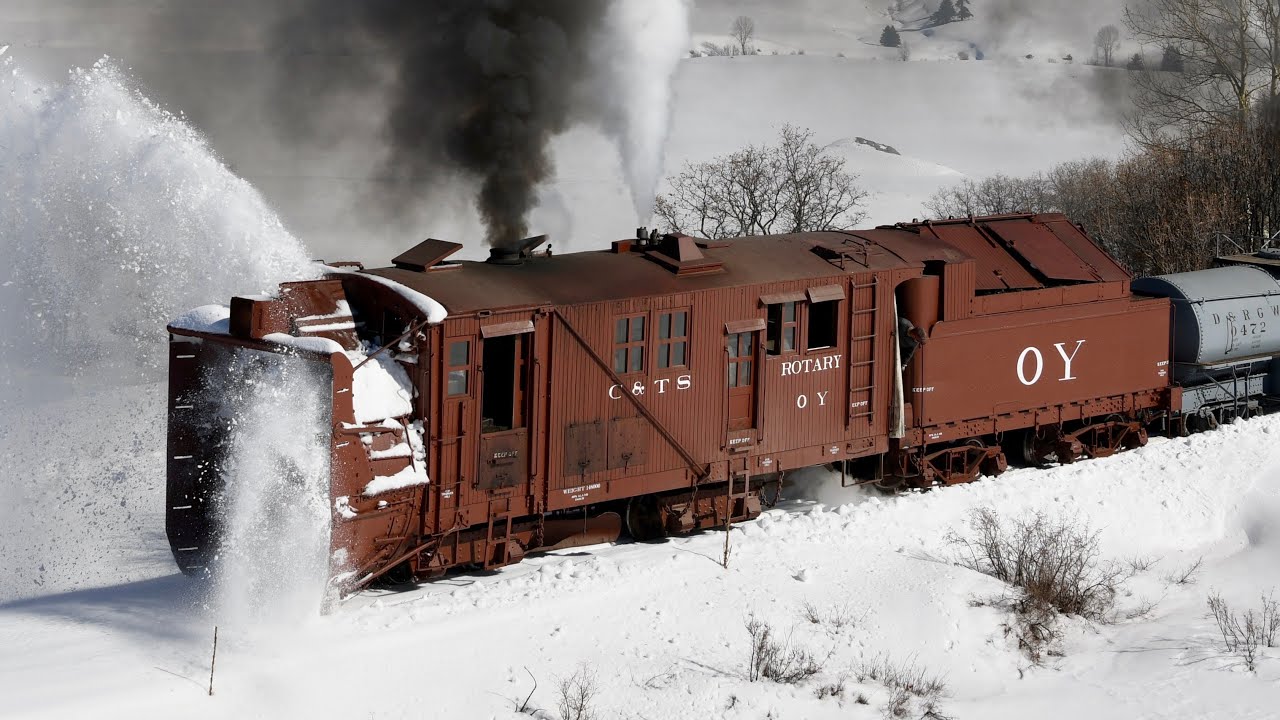In the photograph, a snowplow-equipped train is seen navigating through a snow-covered landscape. The locomotive, a specialized snowblower, features a wide metal apparatus at its front designed to clear snow from the tracks by funneling it into a chamber and expelling it out the sides. This action produces a dramatic spray of snow flying out to the right of the image. The train emits both dark smoke, indicative of a large diesel engine, and white steam, possibly from vents.

The train consists of multiple cars: behind the rusty brown locomotive, there's a gray tanker car likely used for fuel, and a weathered red car. The side of the locomotive bears the marking "CNTS Rotary OY," with "OY" also displayed prominently on the coal car. The setting is a snowy expanse featuring some close trees devoid of leaves and distant tree-lined pastures, suggesting winter's grip. The sun casts shadows on the right side of the train, indicating it might be late afternoon. The scene captures the train's robust effort to clear a path through the heavily encrusted snow-covered railway.